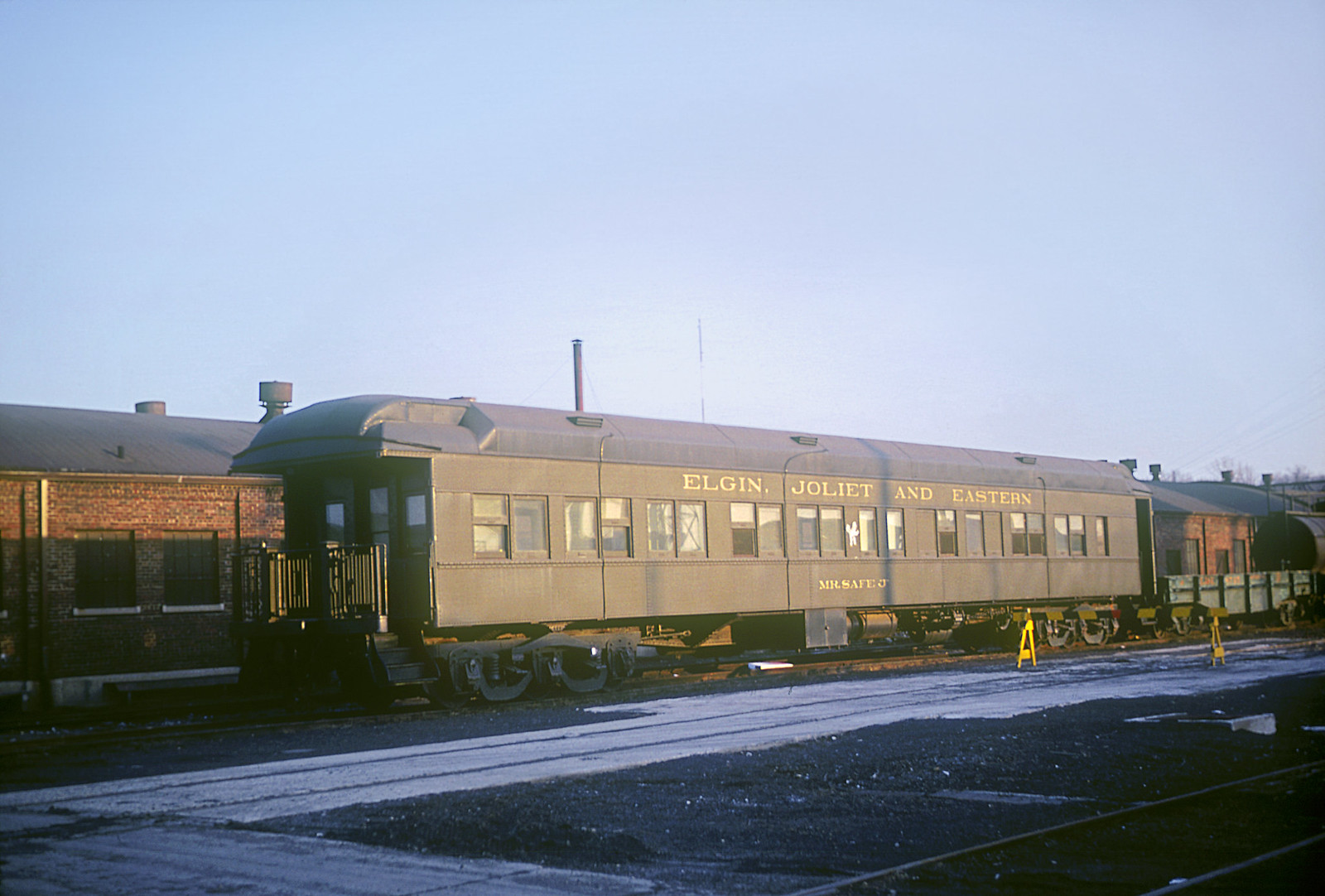This detailed color photograph, taken in landscape orientation, showcases an older gray passenger train car emblazoned with "Elgin, Joliet, and Eastern" in gold lettering across the top. The train car is stationed on a set of rail tracks in the center of the image. To the left end of this car, some metal railing is visible, and an open flat car can be seen behind it. The sides of the train car are light gray, with a blue and purple top. Below and in front of the train tracks, there is a gravelly ground with patches of snow, leading to another set of tracks in the bottom right corner. The scene is bathed in sunlight shining from the right, casting light onto the train car. Above, a hazy, pale blue sky takes up the top half of the picture. Behind the train car, there are two buildings: one is a brick structure, likely a train station, with a couple of windows that might be boarded up, and another is a shorter, wood-toned building with a gray roof. The overall style of the photograph is representational and realistic, capturing intricate details with precision.